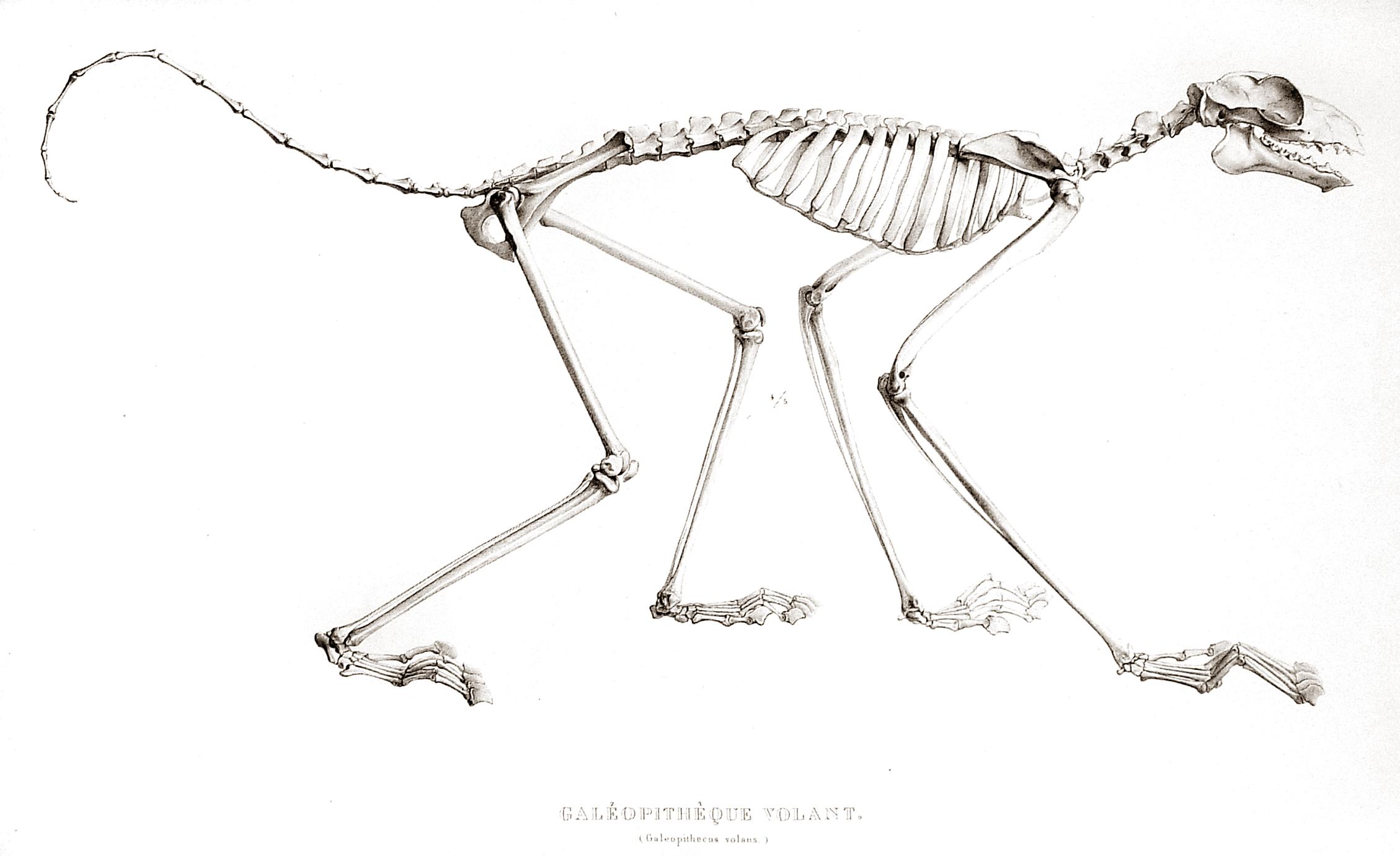This black-and-white illustration presents a detailed skeletal structure of a four-legged animal, resembling a dinosaur or a large mammal, drawn with precision likely using pencil or marker. The elongated skeleton is displayed horizontally from left to right, centrally positioned against a predominantly white background. Notable features include a long tail that extends upward before curving down, a robust back with an articulated spinal cord and rib cage, and a lengthy neck culminating in a sizable head adorned with a long snout and sharp teeth. The skull features a prominent eye socket. The limbs are notably long, ending in what appear to be clawed toes, suggesting an agile, perhaps predatory creature. Below the illustration, there is a line of text in Latin that is difficult to read due to its small size and poor contrast against the background, hinting at the scientific or educational nature of the piece. The image has a slightly faded quality, suggesting it may have been scanned from an original printed document.